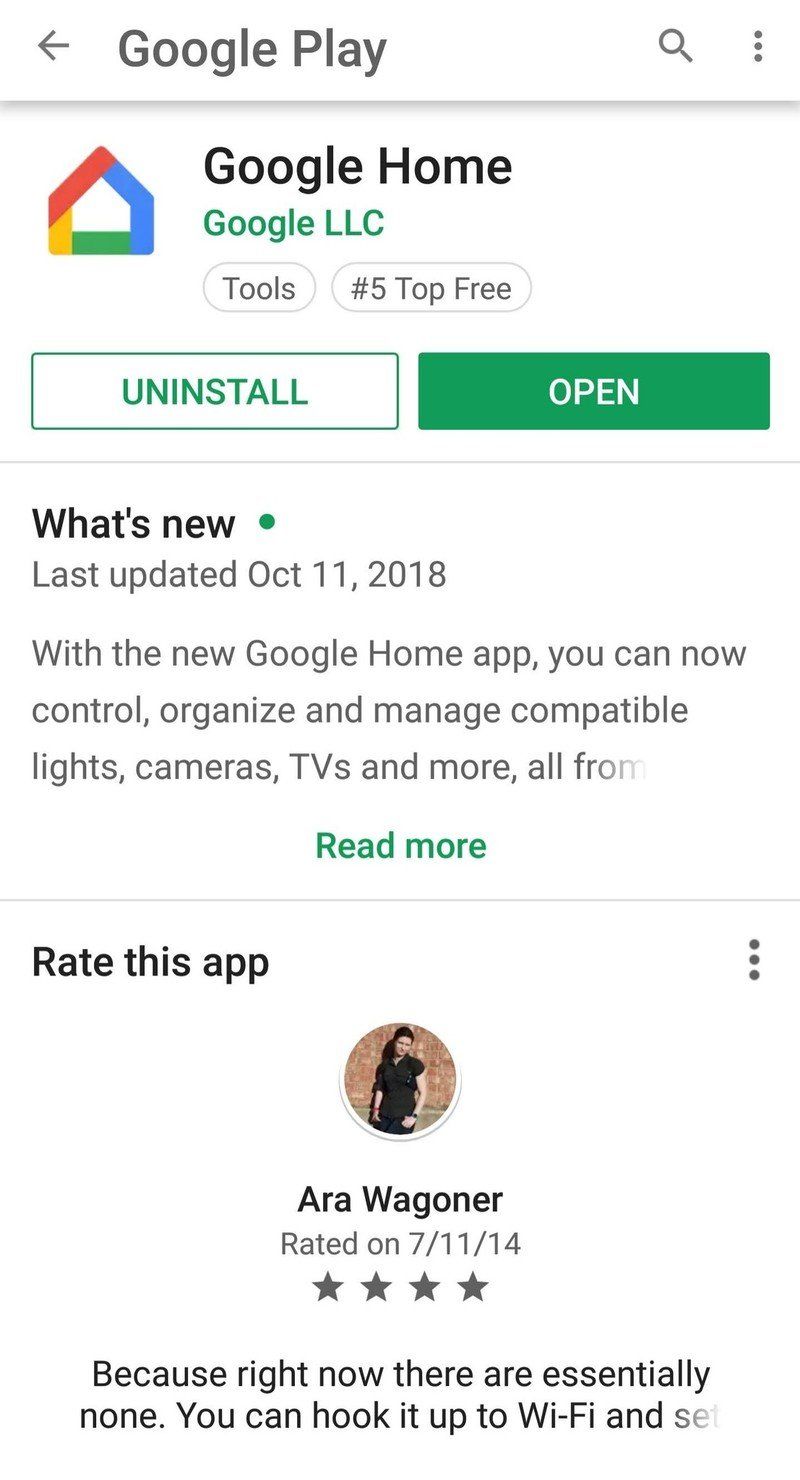In the image captured from a phone screen, Google Play is open, highlighting the Google Home app by Google LLC. The app's icon features a minimalist house design with distinct colors: blue on the right side, green on the bottom, yellow extending up one side, and a red roof on the top left. The app is labeled as a tool and is currently ranked number five among top free apps.

The interface shows a white 'Uninstall' button with green text on the left, and a green 'Open' button with white text beside it. Further down, the "What's New" section indicates that the latest update was on October 11, 2018. The description notes that the new Google Home app allows users to control, organize, and manage compatible lights, cameras, TVs, and more, with a prompt to "read more" in green text for additional details.

The subsequent section invites users to rate the app. A review by Aria Wagoner, dated July 11, 2014, awards the app four stars. The review comments briefly, suggesting limited functionality at the time, before abruptly cutting off.